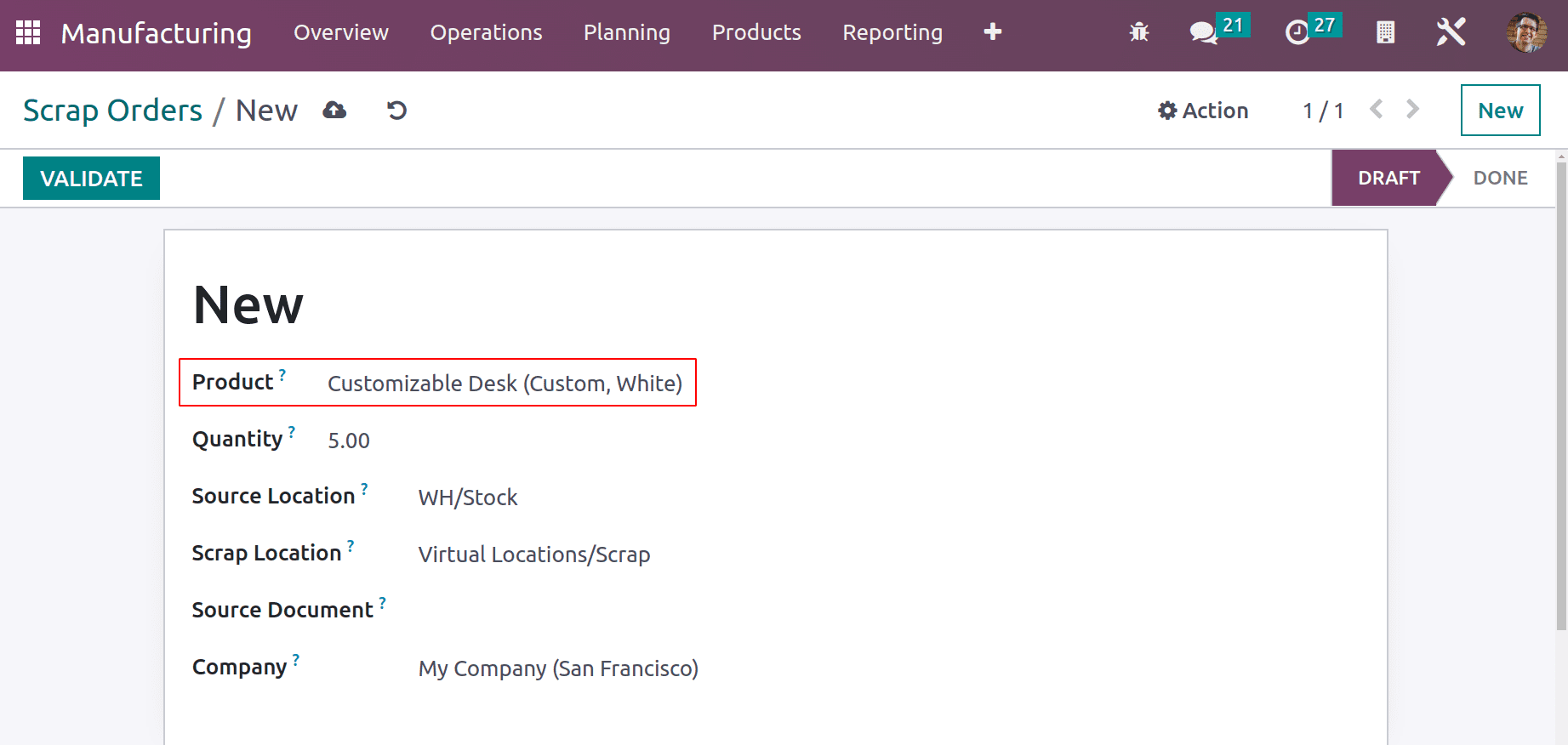The image depicts a detailed view of an interface page. At the top left, there are several navigational links including "Manufacturing," "Overview," "Products," "Reporting," and "Messages (21)." Additional links include "Time (27)" and "Settings." The page features various functionalities such as "Scrap Orders," "New," "Upload," "Refresh," "Action," "Draft," "Done," "Validate," and "New."

The central section highlights a product labeled "Customizable Desk, Custom Bracket, White" within red borders, indicating a selection or alert state. The product's details include a quantity of "5.00" and the source location listed as "WH/Stock." The scrap location is identified as "Virtual Locations/Scrap," and the source document is aligned with a company named "My Company" based in San Francisco.

The interface is set against a purple, green, and white background with black text, while the highlighted sections around the product are marked in red for emphasis.